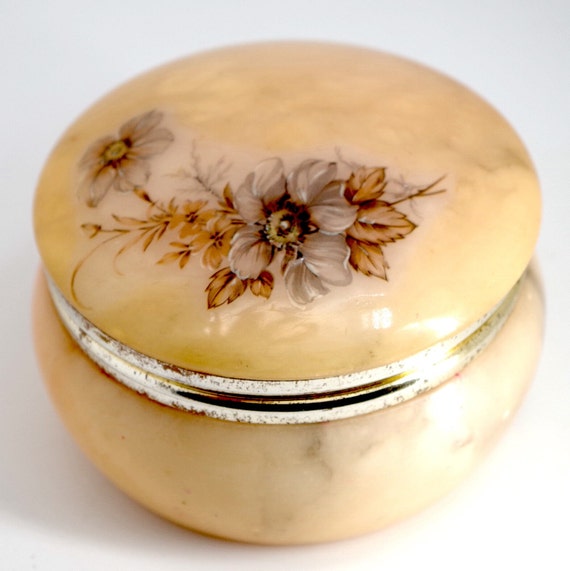This up-close, indoor photograph captures a circular jar, likely intended for makeup or cream, featuring a meticulously crafted, polished marble-like appearance. The jar consists of two sections: a screw-on lid and a lower compartment, both adorned with a decorative gold rim. The exterior of the jar is primarily brown, with the polished finish giving it a luxurious feel. On top of the lid, there’s a detailed illustration of flowers, characterized by brown leaves and petals that transition into light gray or beige tones. The jar rests on a light gray or whitish surface, enhancing its intricate details. Additionally, there is a visible light source coming from the right side, illuminating the jar and highlighting its smooth texture. The background remains unadorned to keep the focus on the jar, which seems antique and possibly used for cosmetic purposes, with some residue of powder adding to its historic charm.